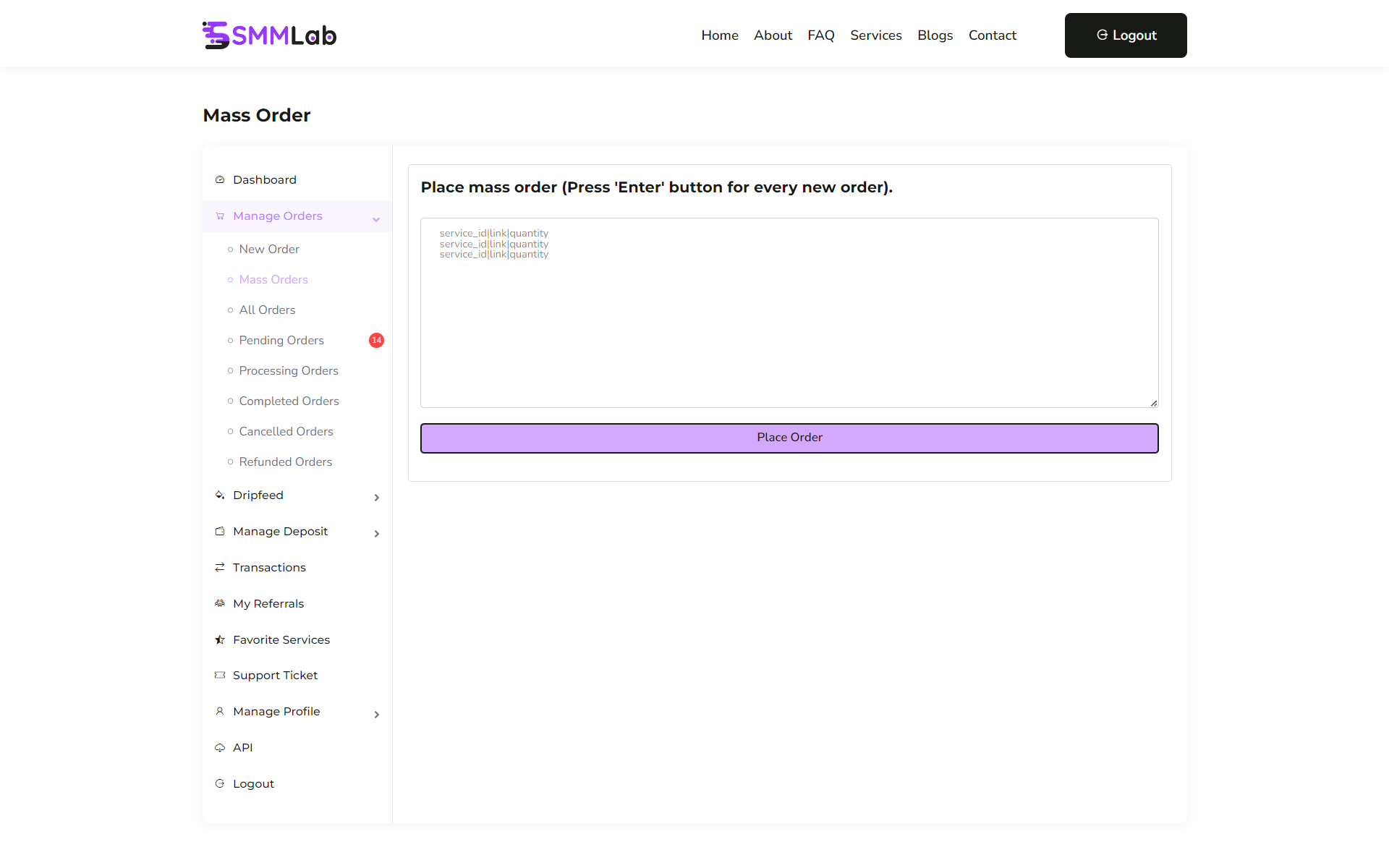The image showcases a color screenshot of a website in square format. The website features a header with "SMM LAB" prominently displayed at the top left, where "SMM" is written in purple, all caps, and "Lab" is in black with only the "L" capitalized. The logo features a stylized "S," transitioning from purple at the top to black at the bottom.

The top navigation bar includes distinctive tabs labeled Home, About, FAQ, Services, Blogs, and Contact. Additionally, there's a prominent black "Logout" button situated at the top right corner.

On the left-hand side of the webpage, there is a vertical navigation menu with several tabs. These include:
- Dashboard
- Mass Order
- Manage Orders, with sub-options: New Order, Mass Orders, All Orders, Pending Orders, Processing Orders, Completed Orders, Canceled Orders, and Refund Orders

Additional tabs on the left menu include Drip Feed, Manage Deposit, Transactions, My Referrals, Favorite Services, Support Ticket, Manage Profile, API, and Logout.

Overall, the layout and design suggest a comprehensive and user-friendly interface typical of service-oriented websites.